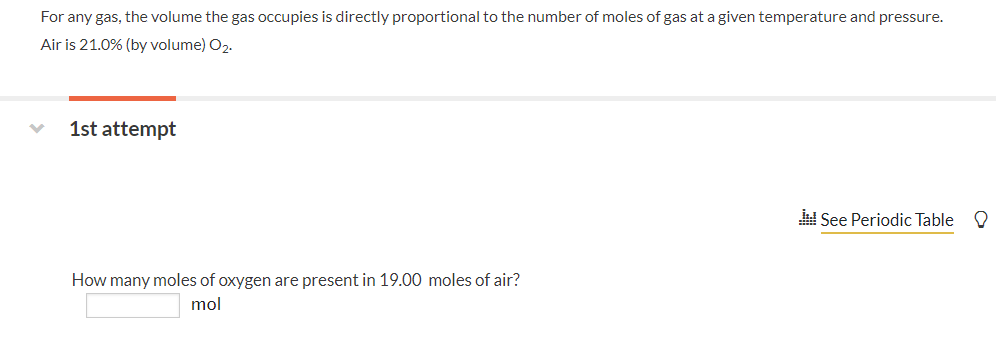In the image, the top left corner features the text: "For any gas, the volume the gas occupies is directly proportional to the number of moles of gas at a given temperature and pressure. Air is 21% by volume O2." Directly below this text, there is a thin, light gray horizontal line extending across the screen, with a segment on the left side highlighted in red. Beneath this red section, the bold, black text "First Attempt" is displayed. To the left of "First Attempt," a light gray downward-pointing arrow is visible.

In the bottom left corner, the question "How many moles of oxygen are present in 19 moles of air?" is presented. Beneath this question, there is an empty white box with "MOL" written to its right. On the far right side of the image, the text "See Periodic Table" is shown, accompanied by a light bulb icon to its right and a graph icon to its left. A yellow line is positioned horizontally beneath the "See Periodic Table" text.